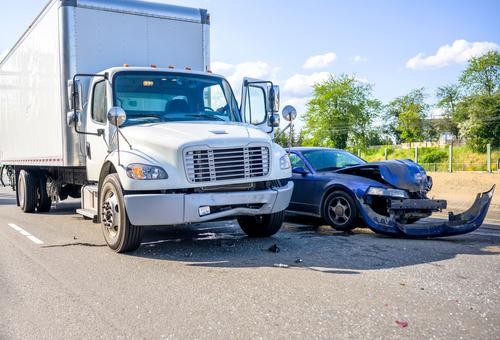The image depicts the aftermath of a vehicular accident on a grey roadway, captured in clear daylight with a bright blue sky and scattered white clouds. On the left side of the image is a large, white boxy cargo truck with its door open and no driver inside. The truck's front bumper is visibly dented. Adjacent to the truck on the right is a severely damaged blue car, with its front bumper completely dislodged and lying on the road, and the hood crumpled in half. The windshield is shattered, leaving glass scattered across the grey asphalt. Both vehicles appear abandoned at the scene. The background features a grassy strip with a couple of trees bearing green leaves, a few bushes, and a sidewalk running parallel to the road. Shadows from the vehicles are cast on the ground, indicating a well-lit setting.